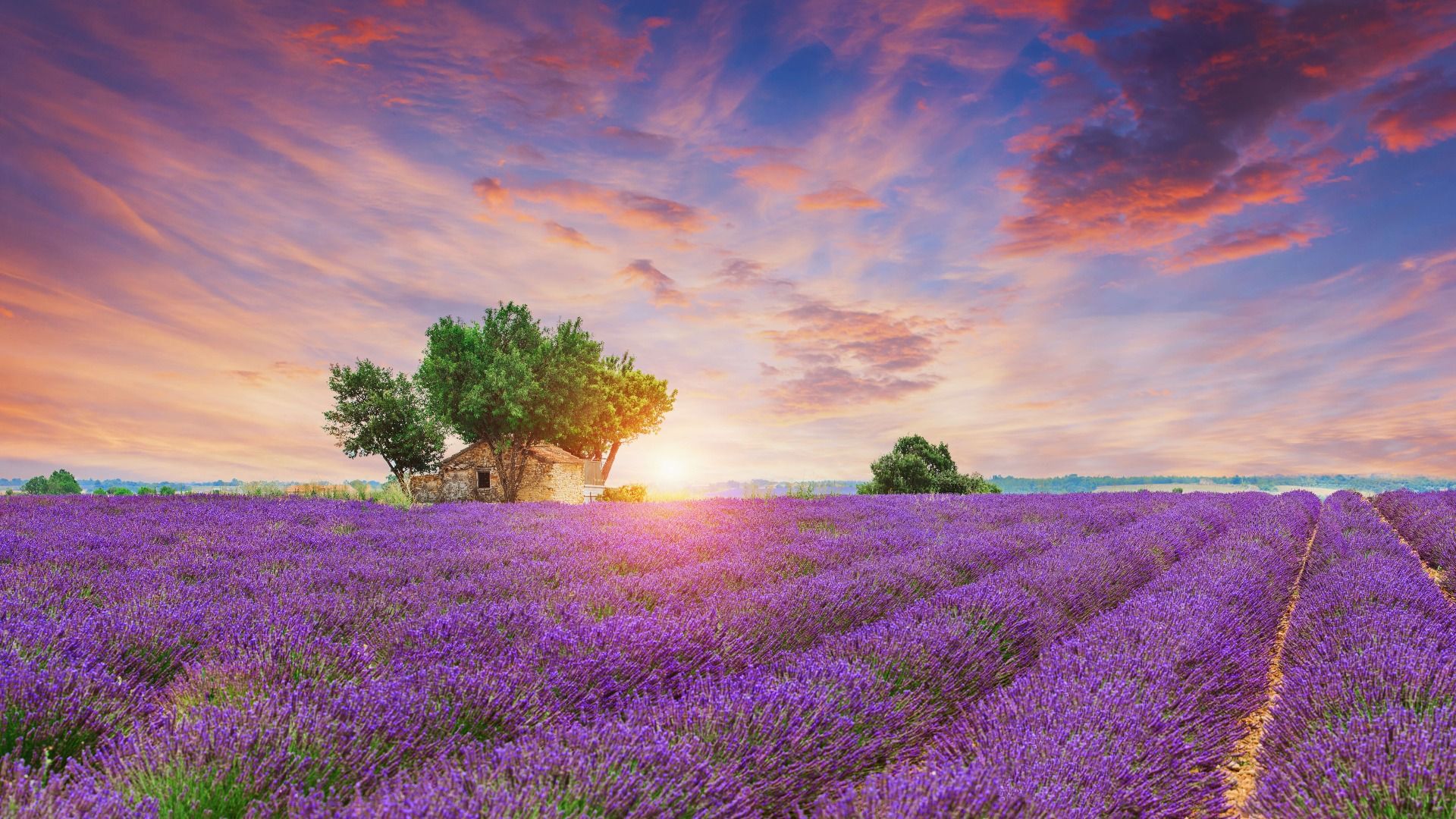The image portrays a stunning, computer-generated scene of a vast lavender field at sunset. Rows of deep violet lavender stretch diagonally across the frame, leading the eye towards the horizon. Dominating the scene, a splendid sunset bathes everything in golden light, casting reddish, pink, and orange hues across the sky and the wispy clouds. To the left of the image, an old stone cottage, surrounded by four or five tall, lush green trees, stands in tranquil solitude. The cottage and trees are softly silhouetted against the radiant backdrop. The sky, taking up about half of the image, exhibits a captivating gradient of blues, pinks, and oranges. The entire scene is imbued with depth, capturing the serene beauty of a summer day as far as the eye can see.